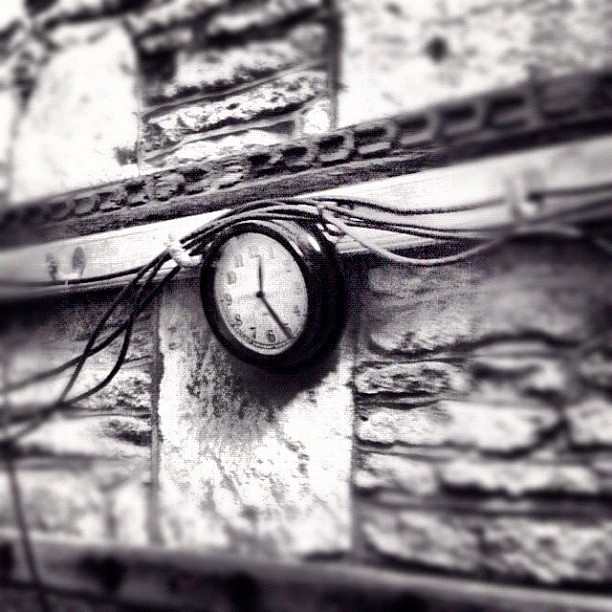This detailed black and white photograph showcases the exterior of a building, distinguished by its intricate stone craftsmanship. The building's facade features a variety of stones, including long, horizontally stacked ones and large capstone-like pieces of limestone or concrete. Small cove moldings, meticulously carved from stone, add to the intricate design. The image also captures flat glass windows embedded in the stonework. Central to the photo is an old-fashioned clock, prominently displayed but precariously tilted forward, seemingly at risk of falling. This clock, with a white face and black numerals, shows the time as 12:25. Surrounding the clock are several wires, supported by metal brackets and hooks, which haphazardly lay over it. The wires and the clock are black, contrasting against the lighter stone surrounding them. Above the clock are scroll-like symbols carved in darker stone. The background includes wood and bricks that are somewhat out of focus, suggesting a layered and aged aesthetic. The mix of materials and the precarious placement of the clock and wiring contribute to the photo's historic and somewhat disheveled appearance.